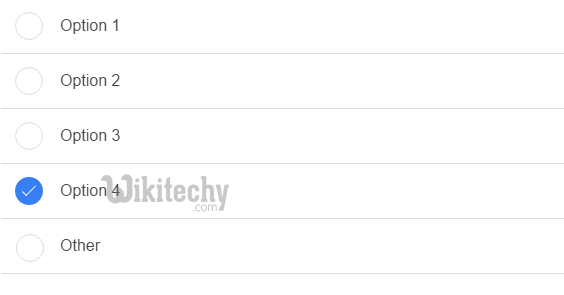This image displays a multiple-choice selection panel with a clean, white background. On the left side of the screen, there are four distinct options presented vertically, each accompanied by a circular selection button to its immediate left. The circles have a light gray outline and a white center. The first option, labeled "Option 1," is at the top, followed by a light gray separator bar. The second option, labeled "Option 2," is below the separator bar. The third option, labeled "Option 3," appears after another gray separator bar. Finally, the fourth option, labeled "Option 4," is positioned at the bottom and is marked as selected, indicating user preference. Each option is separated by a light gray line for clear distinction.